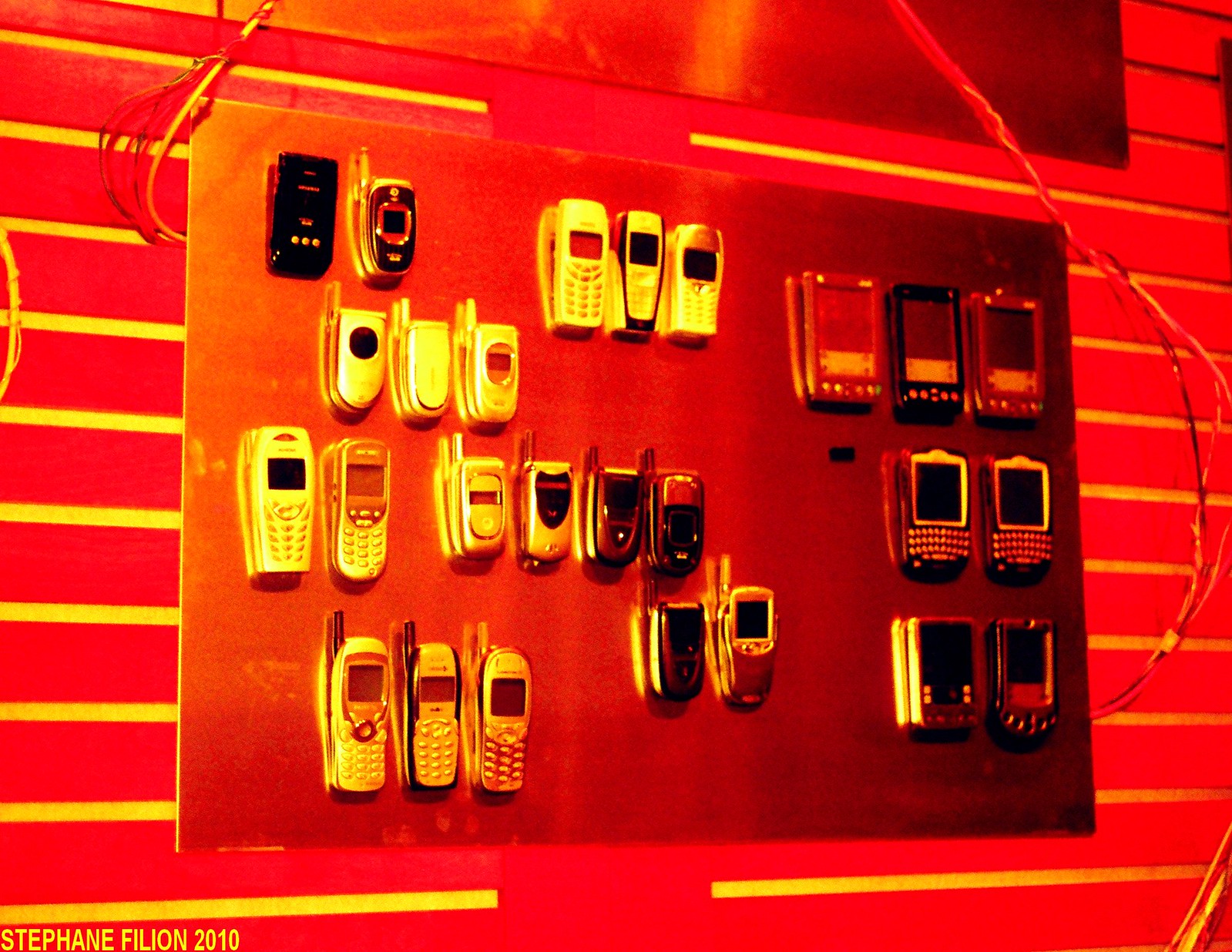This photograph captures a curated display of old cell phones and PDAs, resembling a museum exhibit chronicling the evolution of mobile technology. Arrayed on a metal slab affixed to a wall, the collection features numerous vintage models, including bulky silver phones with darkened screens, classic Nokia phones with prominent antennas, and several flip phones, primarily from Nokia and Motorola. Some cell phones resemble early gaming devices like the Game Boy, characterized by their squared-off designs and minimal buttons. The wall behind the display is vividly illuminated in red with horizontal white and yellow stripes, creating a dramatic backdrop. Additional ambiance is provided by hanging wires draped around the metal slab. The photograph's bottom left corner bears the text "Stephane Philon 2010," further anchoring it in time.